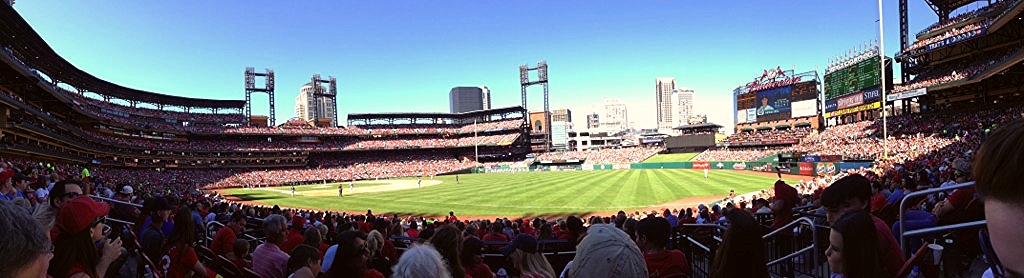This panoramic photograph, taken from the lower levels of a packed, open-air stadium, captures an event on a brilliantly sunny, clear blue sky day. The field, predominantly green, appears to be a baseball stadium. On the far left, there's a distinct dirt area indicative of a baseball diamond, where players are positioned. The right side of the field opens to an expansive grassy area. Rising above the stands, which are teeming with thousands of spectators, are large scoreboards displaying player information. Beyond the stadium, a few tall office buildings punctuate the cityscape, creating a striking contrast with the vibrant blue sky. The sheer density of the audience and their lighter attire suggest a warm, pleasant day.